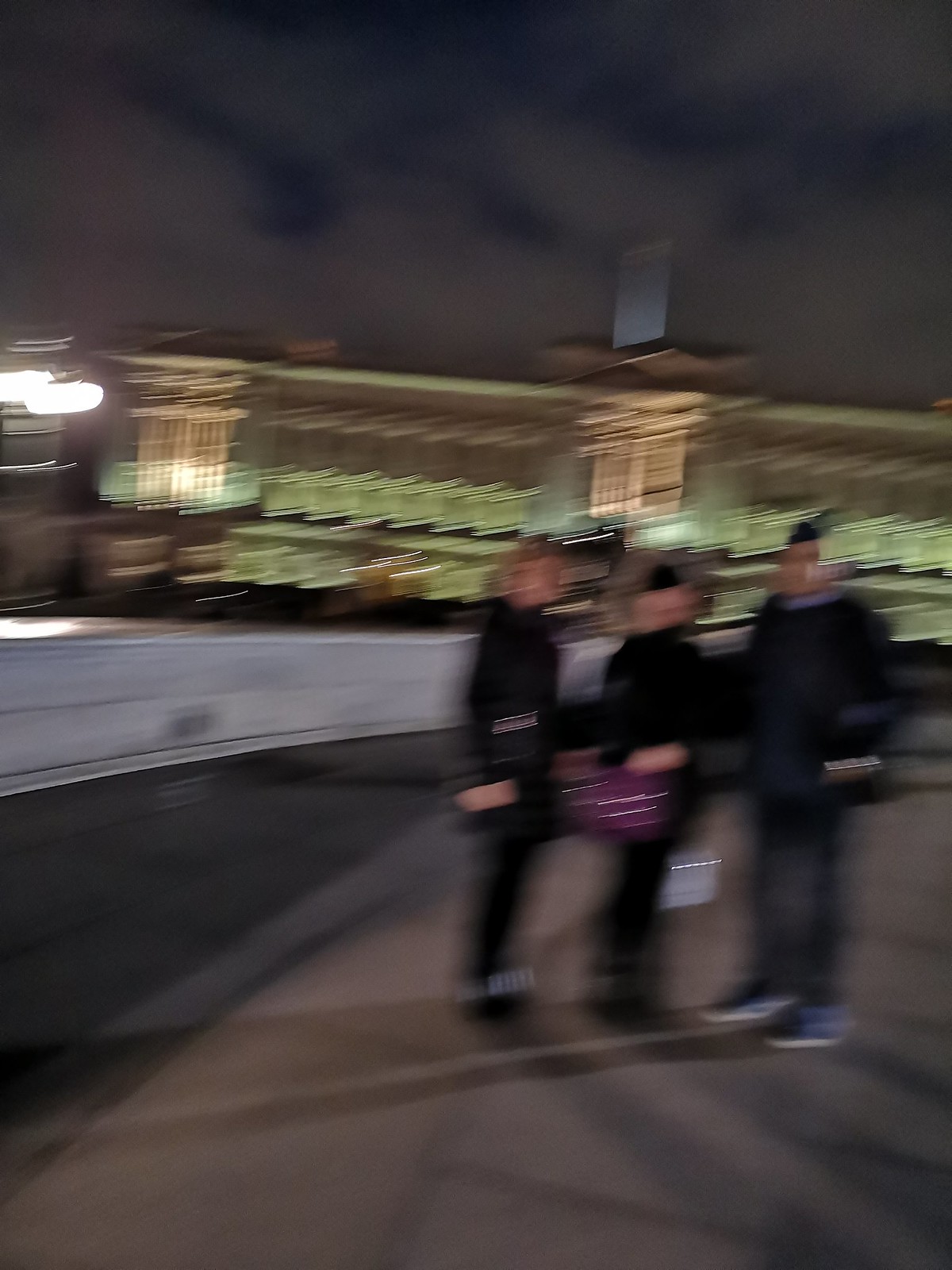This is a blurry, low-quality portrait photograph taken outdoors at night, capturing three individuals standing on a stone walkway. The image appears to be distorted due to rapid camera movement, resulting in a double or triple vision effect. The sky above is a mix of grayish-brown clouds with a hint of remaining daylight and some dark, ominous clouds. In the background, a large, well-lit building with Greek-style architecture, reminiscent of historic European cities like London or Berlin, looms prominently. The building's exterior casts a golden, greenish-brown hue under the low light conditions. 

In the foreground, on the right side of the image, stand three young adults, likely in their 20s or 30s, all with lighter skin tones. They are dressed for cold weather in dark trousers, sneakers, and thick jackets. The person on the far right is a male wearing dark clothes and blue shoes. In the middle is a woman dressed in black, carrying what seems to be a purple purse with silver buttons. On the left, another woman, also in black, has blonde hair and is potentially holding a red bag. Despite their faces being indiscernible due to the blur, all three figures are positioned against the backdrop of this massive, historical structure, making them appear small in comparison to the towering building behind them.